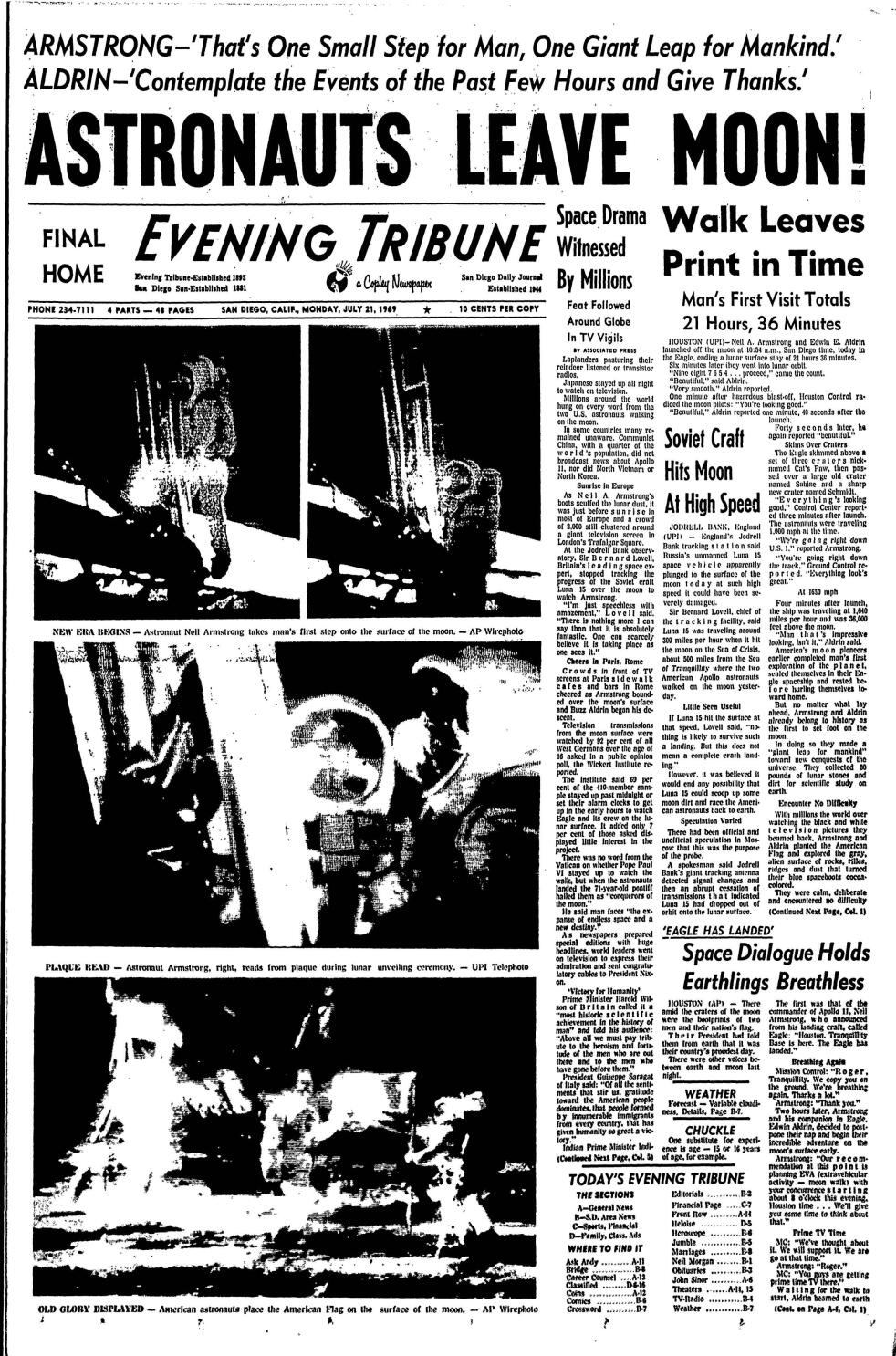The image is a black-and-white newspaper clipping from the 1960s, likely from 1969, documenting the monumental moon landing. Dominating the page, the bold headline declares, "Astronauts Leave Moon." Above this, it commemorates Neil Armstrong's famous words, "That's one small step for man, one giant leap for mankind," alongside a note about Buzz Aldrin reflecting on their journey. The name of the publication, "Final Home Evening Tribune," is prominently displayed, encapsulating the gravity of the historic event. A series of black-and-white photographs on the left side of the page depict the astronauts on the lunar surface, in their spacesuits, planting the American flag. Smaller articles are scattered throughout, covering various aspects of the mission: the total duration of the moonwalk (21 hours and 36 minutes), eyewitness accounts, and the global impact of the event, including a Soviet craft hitting the moon. Captions beneath the photos provide additional context, but the tiny print makes them hard to read. This vividly captures a space drama witnessed by millions, leaving an indelible print in time.